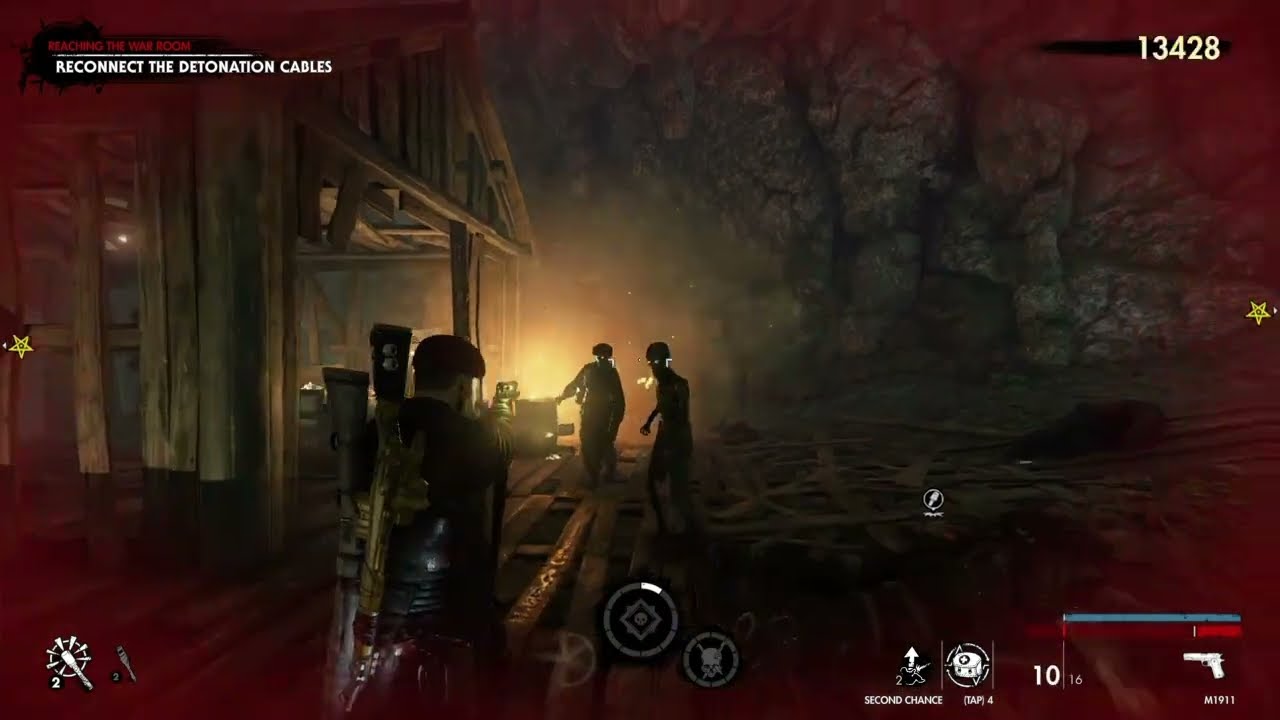This screenshot captures an intense moment in an action-packed, third-person shooter video game. The scene unfolds in a dark, night-time environment resembling a cavern or coal mine, with dim lighting making it hard to discern much beyond the immediate area. The main character, seen from behind, appears male and is armed with multiple guns slung over his shoulder, facing two or possibly three figures ahead of him. These figures, dressed in black uniforms and hats that suggest a soldier-like appearance, might be enemies, possibly zombies given the eerie glow of their eyes. 

To the left, the deteriorating remains of a wooden building or cabin are visible, supported by poles that once held the roof. The ground beneath the characters' feet is strewn with dark-colored wooden boards. In the backdrop, one can faintly make out the contours of trees or rocks, adding to the ominous ambiance.

The user interface elements are prominent, providing crucial information. In the upper left-hand corner, white text instructs to "Reconnect the detonation cables," outlining the player's current mission. The upper right-hand corner displays numbers, likely part of the game’s HUD. In the lower right-hand corner, a HUD shows a gun icon, a health bar, and an energy bar, alongside ammo details, indicating both the type of gun in use and available ammunition clearly.